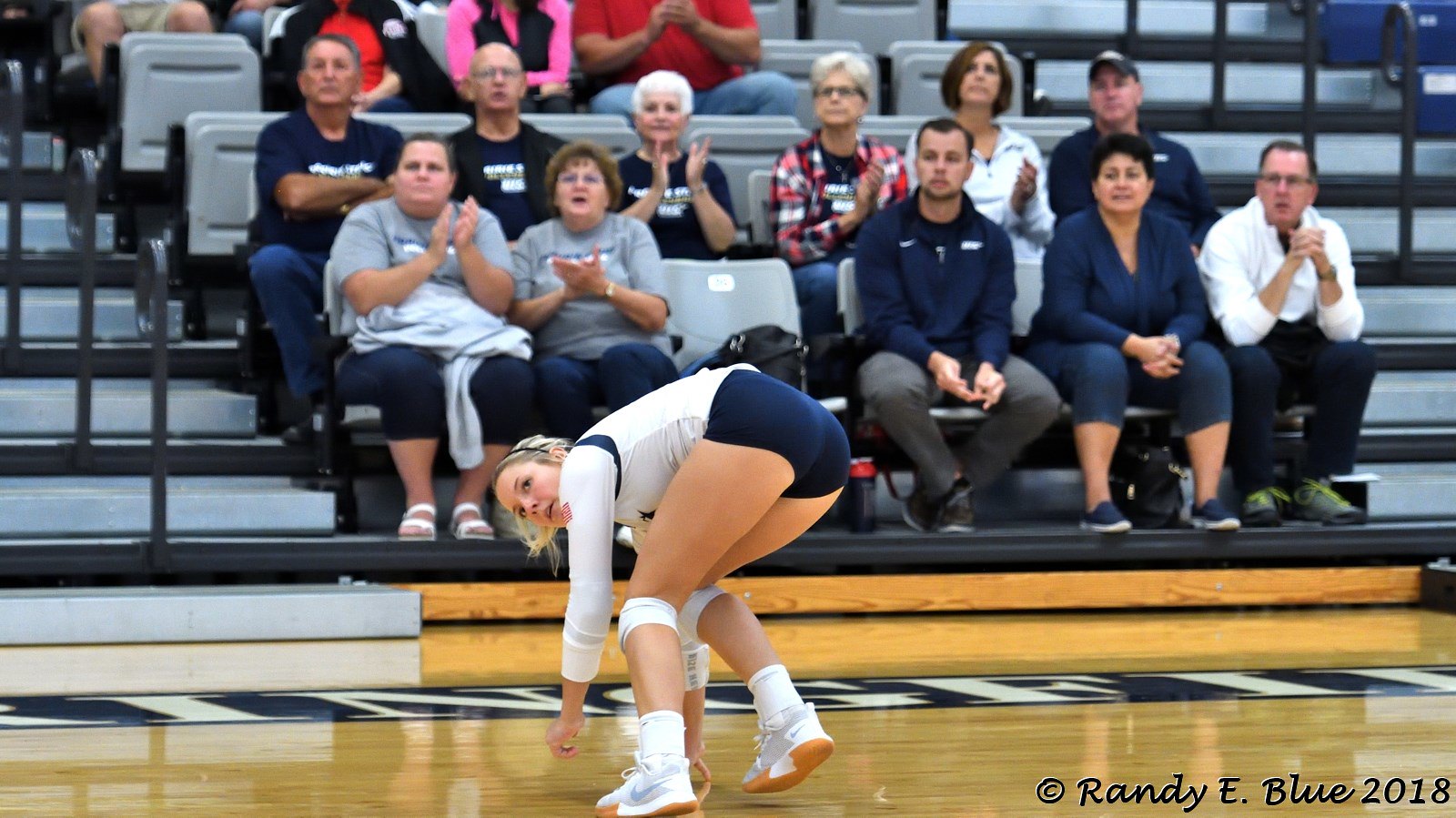This detailed photograph captures a moment during a women's volleyball game, where a white blonde player, dressed in a white and blue long-sleeve shirt and extremely short, tight blue shorts, is prominently featured in the center of the frame. She appears to have just fallen, bending over with her hands touching the gym floor, her rear facing the camera. The scene reveals her white shoes with matching white socks. The background showcases a slightly blurred section of the stands filled with spectators. Among them are predominantly women, some with their arms up as though they're about to clap, and others watching the game intently. These spectators sit on grey fold-open bleacher chairs. The image is complete with a watermark in the bottom right corner that reads "© Randy E. Blue 2018."